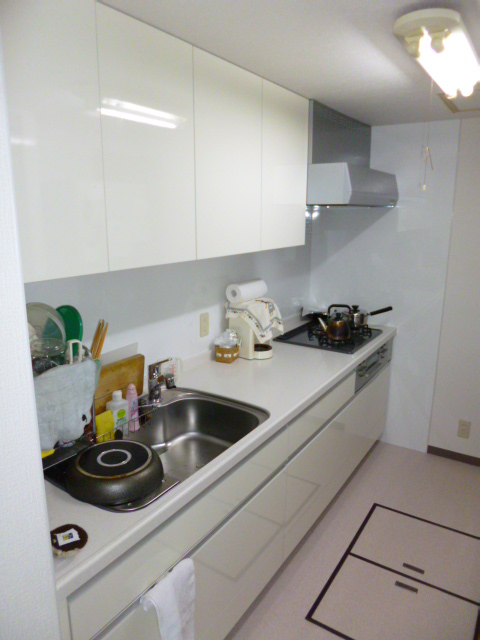A detailed caption for a voice-described kitchen image:

"This image showcases a modern kitchen captured from a cellphone. The kitchen features a sleek design, with both the lower drawers and upper cabinets adorned with a glossy, shiny surface. Dominating the foreground, a metal sink situated on the counter is accompanied by an adjacent drying rack. In this rack, an upside-down frying pan stands out prominently, while additional items such as plastic utensils and possibly chopsticks are drying nearby. A cutting board and a small tray for sponges and various washing implements are positioned behind the sink.

The middle section of the counter remains mostly clear, except for a basket, a covered device with an intricately bordered cloth, and a roll of paper towels balanced atop it. Along the wall is a charging outlet. Towards the back corner of the kitchen, an induction stove hosts a kettle and a pot with its lid on, beneath a vent hood designed to expel smoke. The kitchen is brightly illuminated by overhead fluorescent tube lights.

Adding to the kitchen’s functionality, an additional electrical outlet is visible on the ground in the back. There appears to be underground storage, suggested by two small hatch doors on the linoleum floor. This well-organized and efficiently utilized kitchen space marries practicality with modern aesthetics."